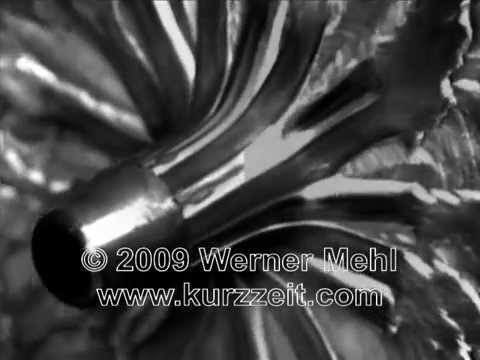This black-and-white photograph, captured by Werner Mel in 2009 (© 2009 Werner Mel, www.curzit.com), features a mysterious and abstract metal object. The image, steeped in various shades of black, gray, and white, presents a flat-bottomed structure that extends into a single, more complex form at the top. It has an artsy, elusive quality, resembling a bottle-like figure or a post with protruding arms, emerging from a dark background. The photo's close-up and slightly out-of-focus nature, combined with the prominent copyright text, further enhances the enigmatic and intriguing appearance of the object.